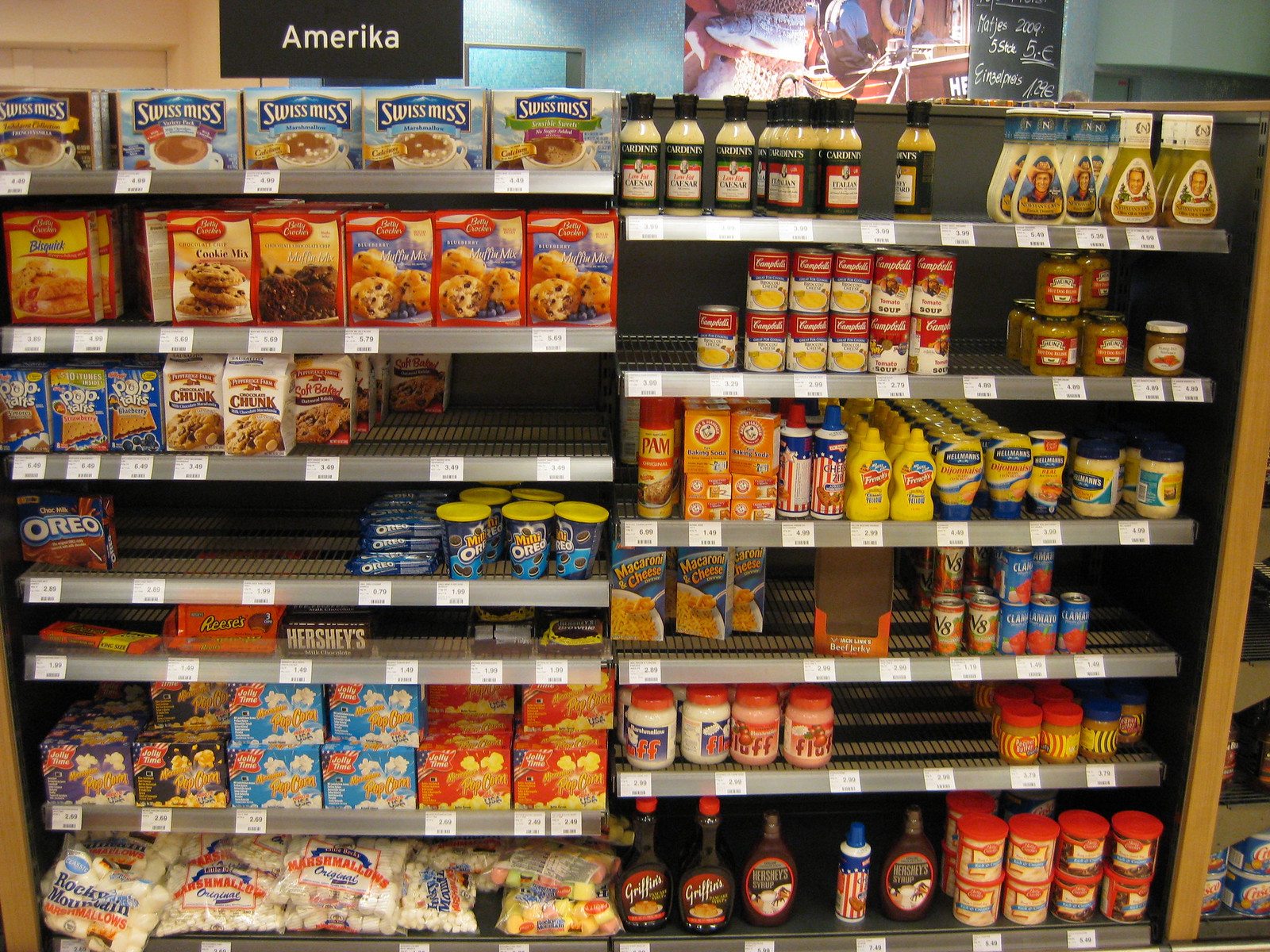The image depicts a grocery store aisle with six shelves, filled with a variety of food products. At the top of the shelves is a black sign displaying the word "Amerika" in white text. The left-hand column showcases snack foods and easy-bake items, starting with Swiss Miss at the top, followed by cake mixes, Pop-Tarts, cookies, Oreo packets, chocolate bars, popcorn, and marshmallows. On the right-hand column, there are sauces, condiments, and spreads, including dressings, jars of various sauces, soups, Pam non-stick spray, canned cheeses, mustards, mayonnaise, macaroni and cheese, juices, pancake syrup, chocolate syrup, and frosting cans. A blue wall with a large advertisement is visible in the background along with some green and brown elements surrounding what appears to be a door.